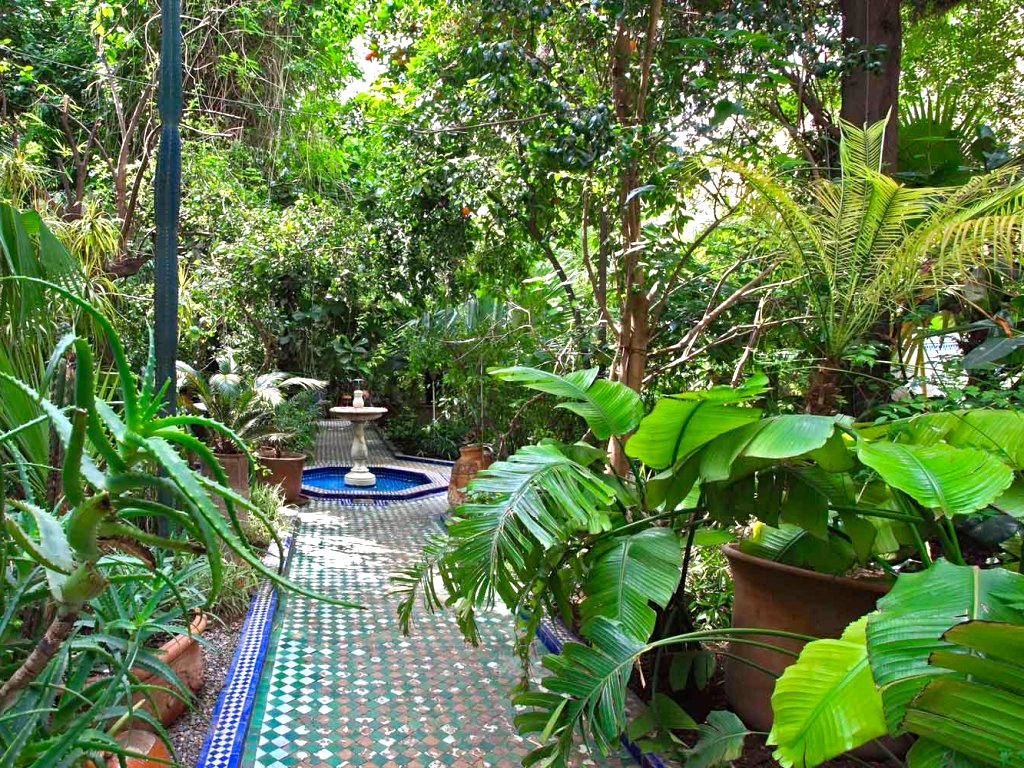This vibrant image, in landscape orientation, captures a peaceful and lush garden scene featuring a central trail leading to a fountain. The trail, starting at the bottom of the photograph, is paved with intricate blue, white, and reddish tiles, accented by a darker blue-tiled raised section on either side. The central fountain, midway through the image, boasts a single tier atop a pool of dark blue water, with a little white structure emerging from it. The garden teems with greenery; to the left, tall plants including aloe and other tropical varieties dominate, while the right side showcases large terracotta planters filled with philodendrons, ferns, and more flora. Overhead, mature trees provide ample shade, allowing dappled sunlight to filter through. Small details such as electrical lines at the top of the image peek through the dense foliage, adding modern touches to this serene, nature-filled setting. The scene is rendered with photographic realism, truly capturing the tranquility and beauty of the environment.